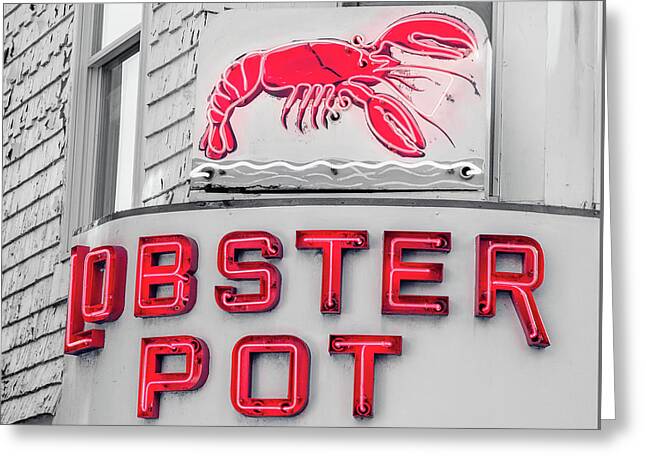The image features the front of a restaurant on a gray building with distinct vertical sections resembling shakes. Prominently displayed is an LED neon sign for the "Lobster Pot," centrally positioned and composed of capitalized red letters with a white neon outline. Above the text is a realistic red lobster, oriented with its claws to the right and its tail curved downwards on the left. The lobster is further detailed with white and black outlines, adding depth to its appearance. The sign, resembling a cylinder with two layers, is adorned with wavy lines beneath the lobster, likely representing water and contributing to the artistic feel of the scene. Off to the left, the textured building wall extends to a standard closed window, while the right side of the image remains a plain gray background, emphasizing the vivid red of the restaurant's sign and the lobster against the otherwise monochromatic setting.